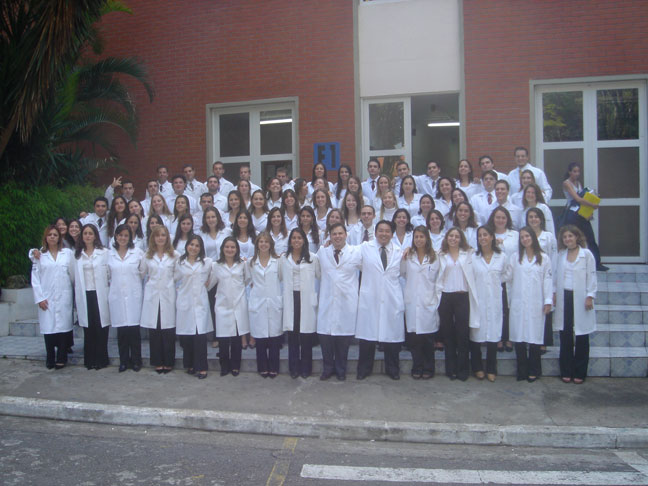This vibrant color photograph captures a large group of medical students in their pristine, long white lab coats during a white coat ceremony. The group, consisting of both males and females, is arranged in five rows on the steps of a red brick building, likely a medical facility, as inferred from the professional attire and setting. The building boasts wide windows with six panes on each side and an open door at the top of the stairs, with some tropical-looking shrubbery and palm-like trees adding greenery to the scene. The students, dressed professionally with black and brown leather loafer-like shoes, are smiling broadly, embodying the joy and prestige of the occasion. The background reveals a concrete floor and a parking lot line, while a solitary student, casually dressed in a tank top and carrying a textbook, walks on the steps, adding a touch of everyday campus life to this celebratory image. The building façade is marked with "F1," grounding the scene in a specific, yet unidentified, location.